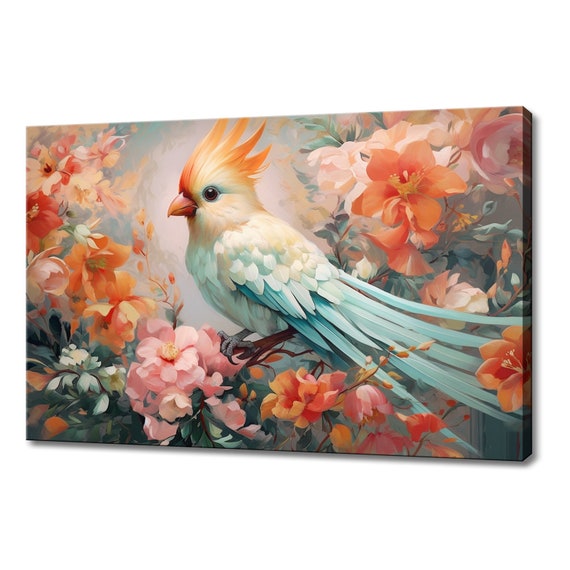The image showcases a professional and vibrant oil painting on canvas, set against a pristine white background. The painting features a colorful tropical bird, believed to be a cockatiel, prominently displayed in the center. The bird is perched on a branch and is oriented towards the 8 o’clock position. It has a striking teal chest and tail feathers, a white back, and a yellowy-white head adorned with an orange mohawk-like crest that resembles fire. The bird's eyes are highlighted with blue eyeshadow, adding to its vivid and lifelike appearance. Surrounding the bird are a variety of blooming flowers in harmonious shades of pink, orange, and blue, enhancing the overall symmetry and balance of the composition. The painting's details, from the bird's mid-life plumage to the colorful floral arrangement, accentuate the craftsmanship and artistic quality of the piece.